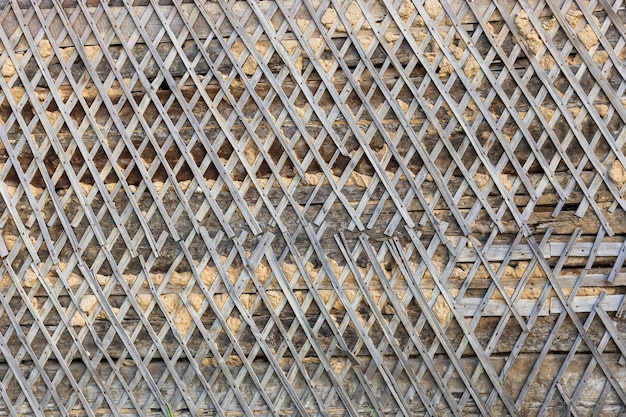The image depicts a detailed photograph of a vertical, crisscross lattice fence made of thin wooden strips arranged in a diagonal, diamond-shaped grid pattern. Each strip is interwoven, creating a densely hatched design with approximately 30 strips intersecting diagonally from the top left to the bottom right, and another set from the top right to the bottom left. The wooden lattice, light brown in color, is broken and missing pieces in several sections, particularly towards the middle and bottom right. This wooden structure is affixed to a robust background comprised of a stone and cement wall, with some areas backed by wooden boards. An unusual yellow, sticky substance appears to be seeping through parts of the grid, suggesting an adhesive might have been used in the construction or repair of the fence. The entire scene is outdoors, with no additional elements or text present in the image.